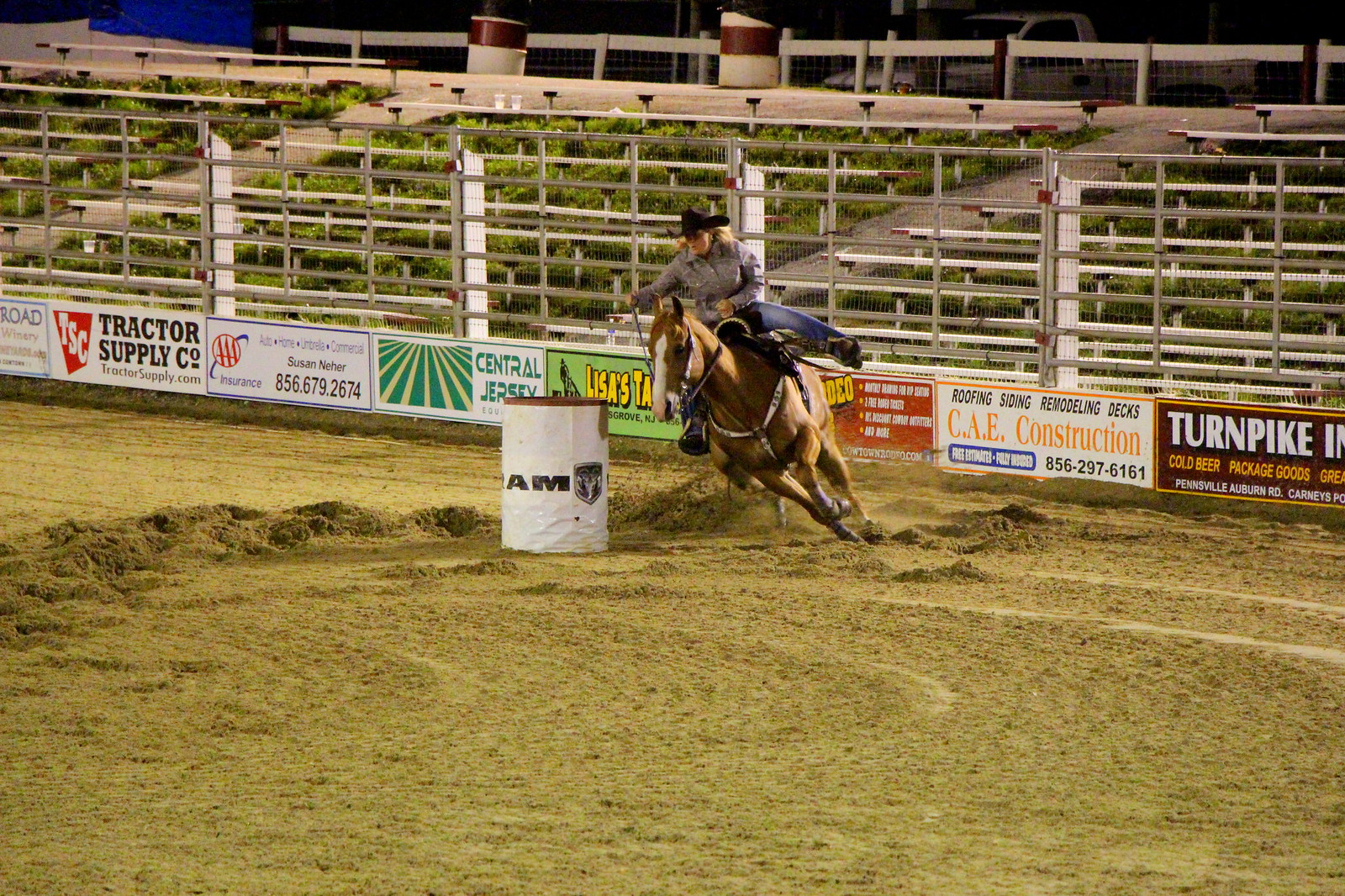In this dynamic rodeo practice scene, a rider with long blonde hair, wearing a grey long-sleeved shirt, blue jeans, and a black cowboy hat, is expertly maneuvering a brown horse around a white cylindrical barrel marked with the letters “AM.” The well-groomed horse, identifiable by the striking white patch on its forehead, gallops across a ground covered in brown soil, leaving visible hoof prints in its wake. Encircling the practice area, a metallic fence adorned with numerous advertisements from local businesses, including a prominent sign for “Tractor Supply Company,” separates the action from the empty bleachers and patches of grass beyond. The photograph captures the intensity and motion of the rider's turn in front of this vibrant backdrop of colorful signs and the rural rodeo setting.